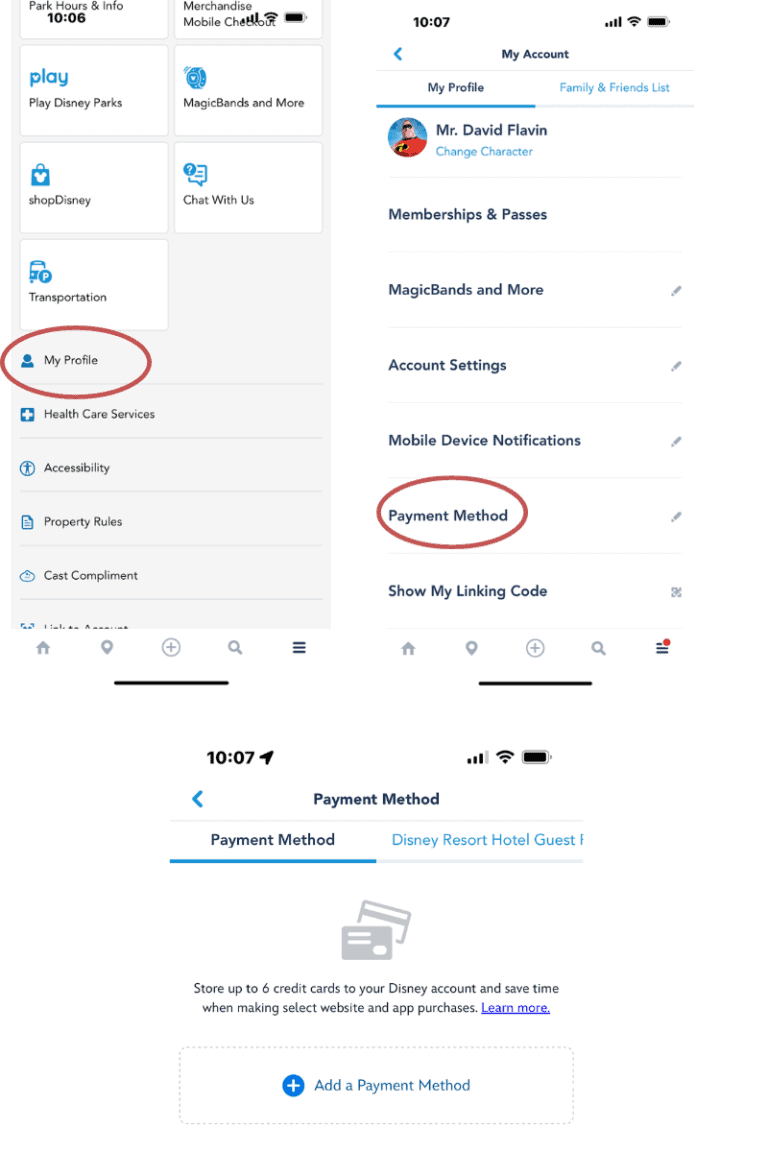The image displays two side-by-side screen captures from mobile devices.

**Left Screen Capture:** The screen is predominantly white with various icons accompanied by their labels. In the center, the "My Profile" icon stands out as it is circled in red. Directly below it are icons for "Health Care Services," "Accessibility," "Property Rules," and "Cast Complements."

**Right Screen Capture:** Similarly featuring a white background, this screen shows the time "10:07" at the top. Beneath the time, the text "My Account" is prominently displayed. Below "My Account," the "My Profile" section is highlighted with a blue underline. A profile image featuring a cartoon character in red against a blue circular background is visible below the blue line.